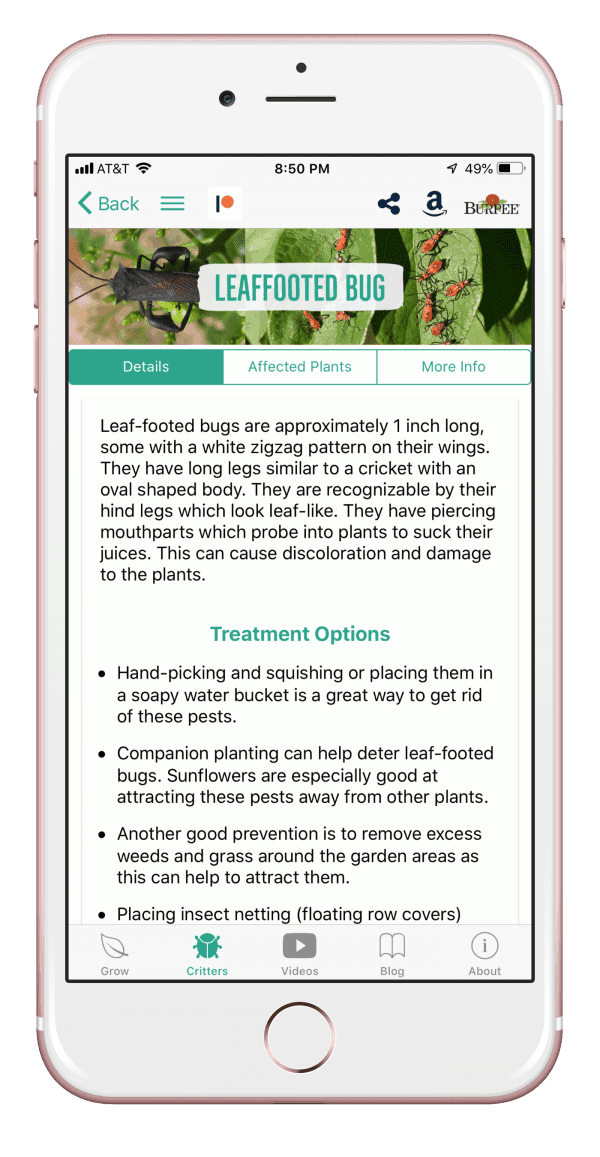The image displays an older model iPhone, possibly from the 7 or 8 series, showing the time as 8:50 PM. The device has full network signal strength, as indicated by 4 out of 4 bars, and is connected to the AT&T network. The battery percentage displayed is critically low at 9%. The text on the screen discusses leaf-footed bugs, which are approximately one inch in length and can be identified by a distinct zigzag pattern on their wings. These bugs possess long, cricket-like legs and an oval-shaped body; their hind legs resemble leaves. They have specialized mouthparts for piercing plants and extracting their juices, leading to plant discoloration and damage. The text also mentions treatment options for dealing with these pests.